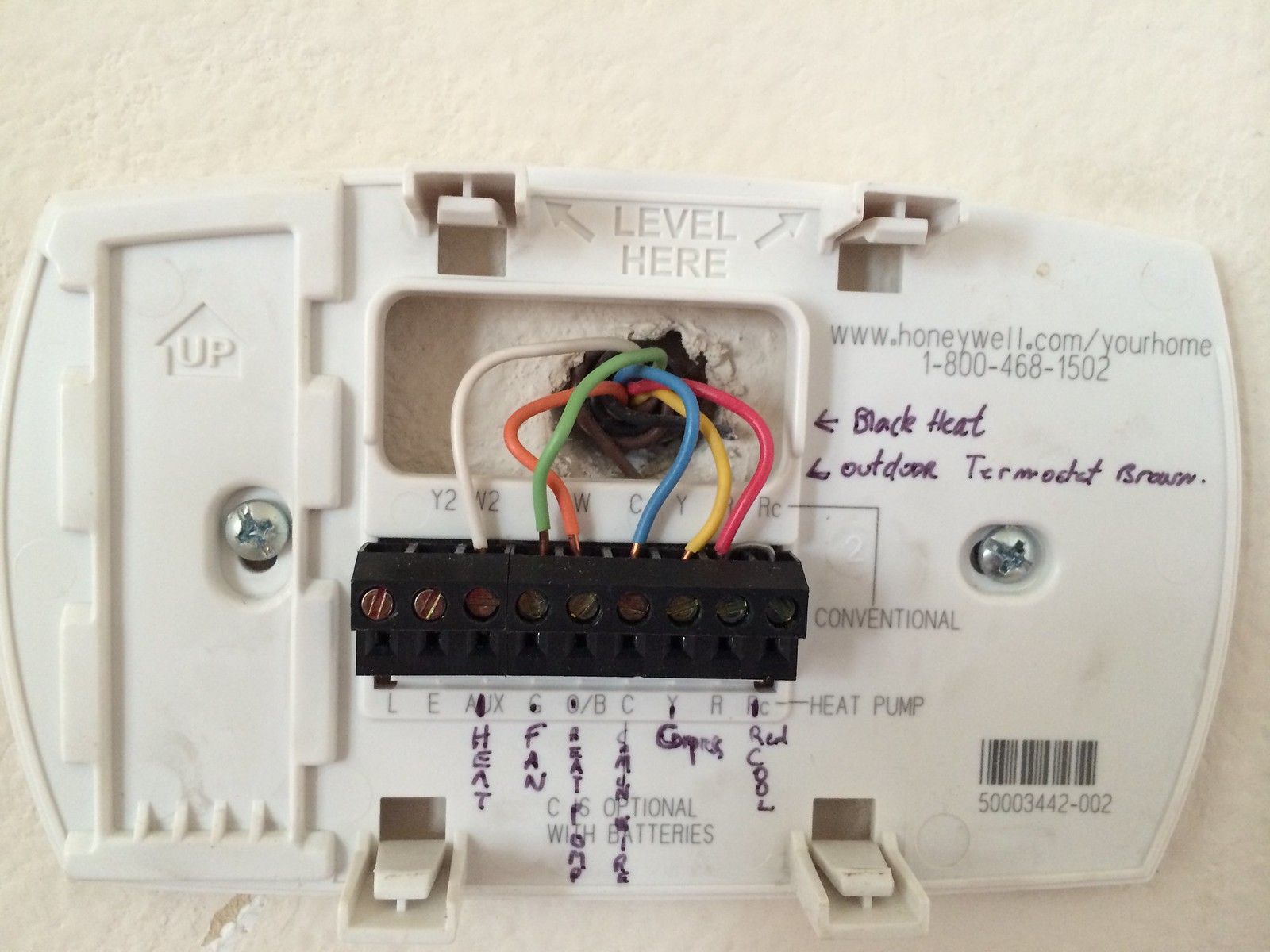The image shows the exposed back of a detached thermostat, which has been removed from its original mounting on a white drywall surface. The thermostat casing is primarily white plastic with factory-printed black text, supplemented by handwritten notes in black ink.

At the top portion of the thermostat's back, the word "LEVEL" is printed, flanked by arrows pointing upward and outward. The base of the exposed thermostat reveals an array of multi-colored wires—white, orange, green, blue, yellow, and pink—protruding from the wall and connecting to a small black rectangular terminal block. This terminal block, equipped with several tiny screws, secure the wires in place.

Prominent within the image are two silver Phillips head screws that secure the thermostat to the wall. Additionally, handwritten labels in black ink identify various components and wiring functions, including annotations such as "black heat" with an arrow and "outdoor thermostat broom brown" with another directional arrow, providing further context for the thermostat's connections and functionality.